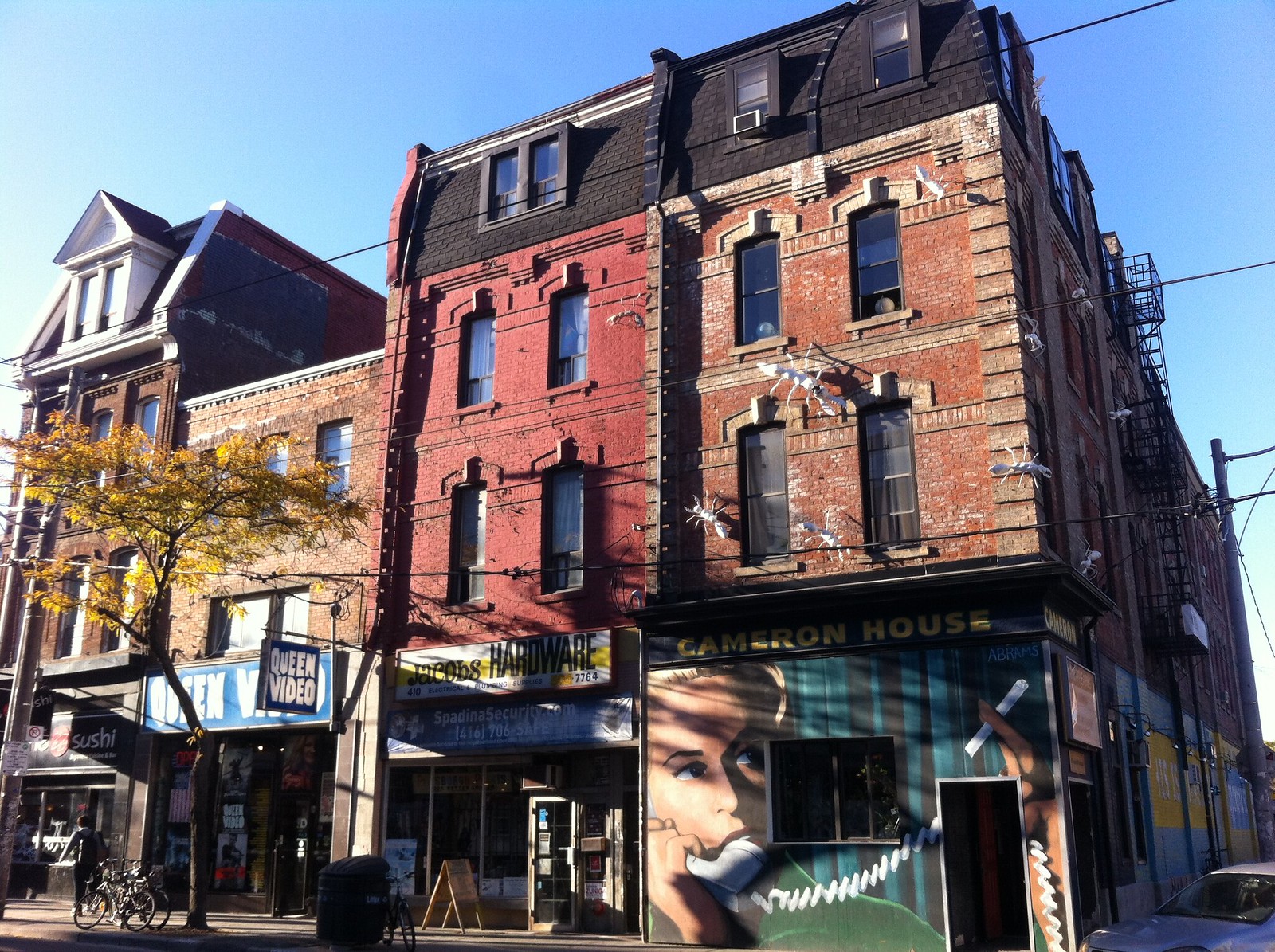The image captures a detailed urban street view featuring four distinct buildings. On the far right, a faded brick building stands out with a mural showcasing a woman holding a white phone and a cigarette, labeled "Cameron House" in yellow letters. Beneath this building, the partial view of a white car is visible. Adjacent to Cameron House is a painted red building housing "Jacob's Hardware," marked by an exterior sign and accompanied by a bag leaning against a mailbox and an advertisement board set up on the sidewalk. Moving left, a shorter faded brick building hosts "Queen Video," distinguished by its white-lettered sign on a light blue background wall. The fourth structure, composed of normal-colored brick, features a sign reading "Sushi." The scene is enriched by a person standing near a utility box in the bottom left corner, all under a mainly clear sky with hues of blue, red, and brown. The architectural composition shows varied heights, with the two rightmost buildings being identical in height and roof design, the third building shorter, and the fourth building matching the height of the first two but with a different roofline.